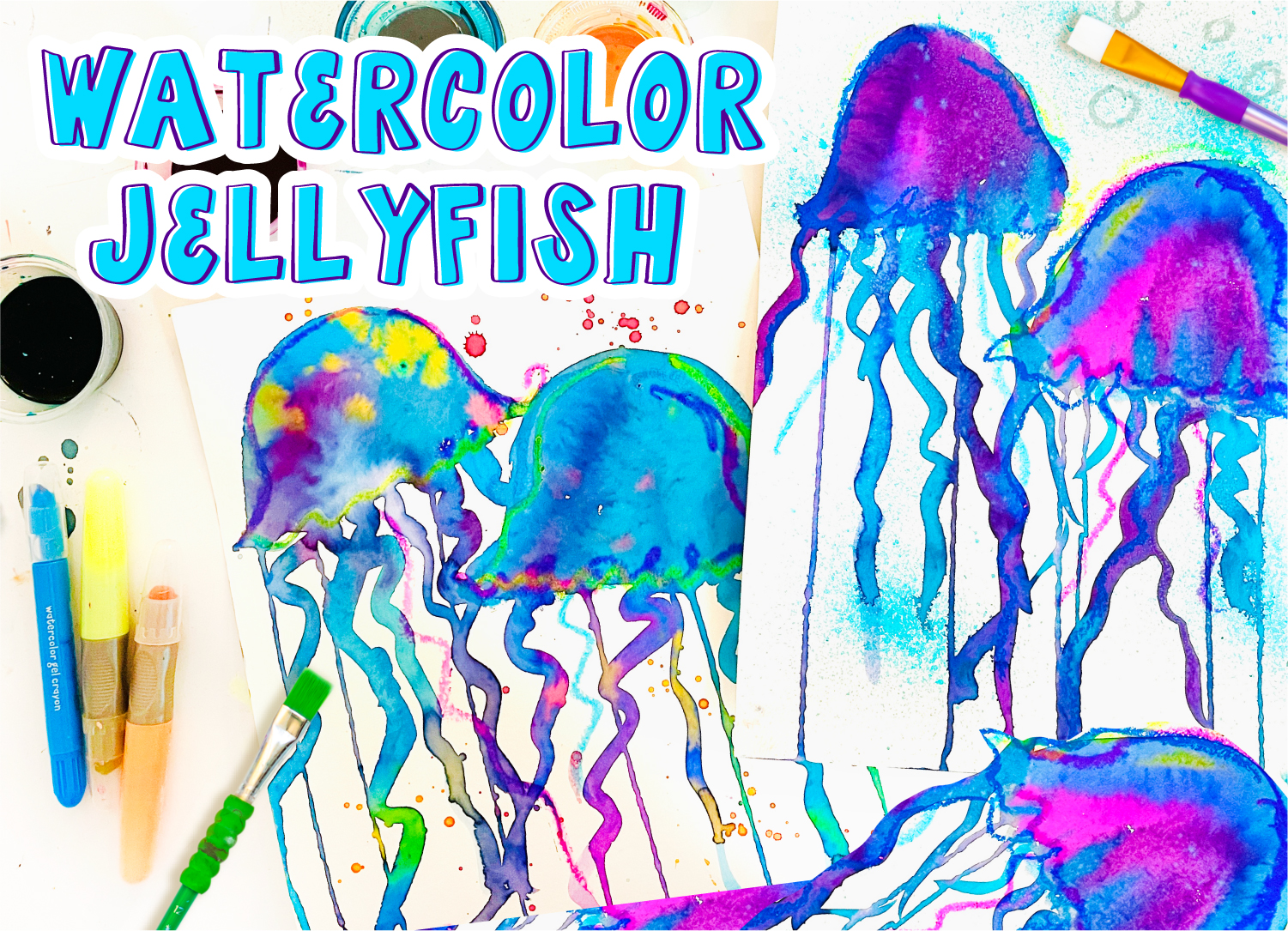This image depicts a vibrant and colorful artistic setup, showcasing multiple sheets of white paper with watercolor paintings of jellyfish, primarily in shades of blue, purple, green, yellow, and pink. The scene is set on a white art table, photographed from a top-down perspective. Scattered around the table are various art supplies, including a white paintbrush with purple and yellow paint, a green-handled paintbrush, markers, and pens in colors like blue, yellow, and green. In the upper left corner, the words "Watercolor Jellyfish" are prominently displayed in large blue letters with a white background and a purple border. A white cup filled with a dark liquid, possibly used for rinsing brushes, is located at the center left. There are splatters and drips of paint around the artwork, indicating the creative process. The entire scene captures the dynamic and lively atmosphere of an artist's workspace.